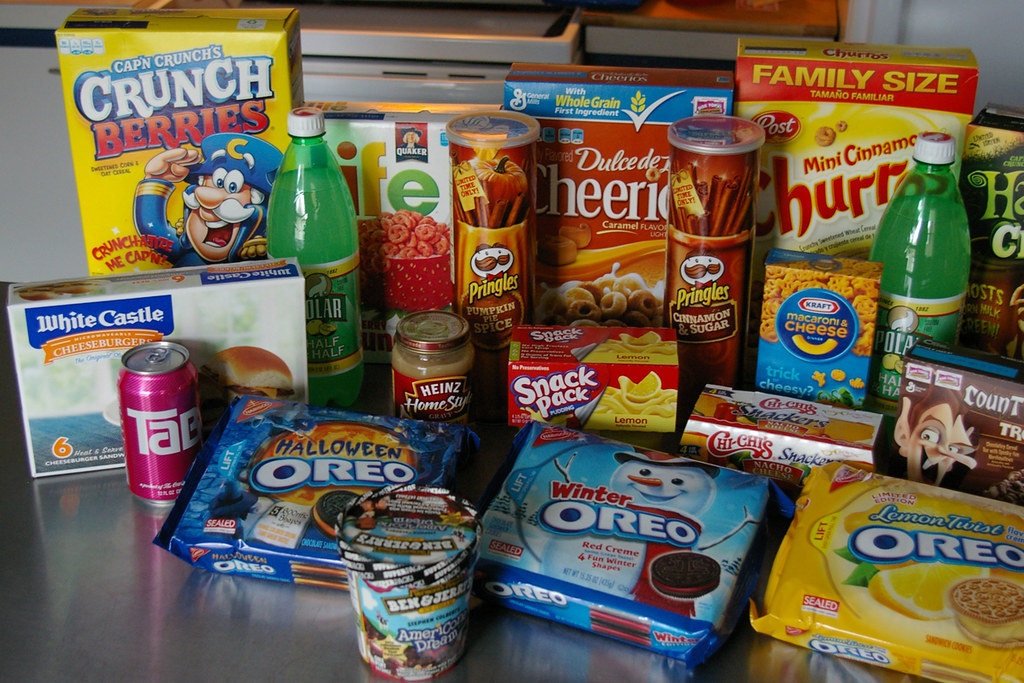The photograph depicts a silver island countertop laden with various grocery store food items, reminiscent of a well-stocked shopping cart. Dominating the upper left, there is a vivid yellow box of Captain Crunch Crunch Berries with the iconic captain character. Adjacent to this colorful cereal box is a muted white box of Life cereal, marked with a vibrant bowl of cereal on its front. Flanking these are multiple boxes and cans: blue boxes of caramel-flavored Cheerios and yellow family-sized Mini Cinnamon Churros, with red and orange cans of Pringles revealing flavors like original and cinnamon-sugar. A pair of soda bottles also make an appearance towards the sides.

Lowering the gaze, one notices a white-colored box of White Castle cheeseburgers, with an assortment of Oreos taking center stage just ahead. There's a trio of special edition Oreo cookies—Black Halloween Oreos with orange cream, Winter Oreos adorned with a snowman and filled with red cream, and Lemon Twist Oreos featuring blonde cookies with yellow cream.

Prominently in front of the desserts, a pint of Ben & Jerry's American Dream ice cream awaits indulgence. Additional items fill in the gaps: a pink can of Tab soda, a brown box with Dracula imagery, Chi-Chi's salsa containers, Heinz Home Style Gravy, a snack pack of lemon pudding, and a box of Kraft macaroni and cheese. Each item combines to create a vivid tableau typical of a family's grocery haul.